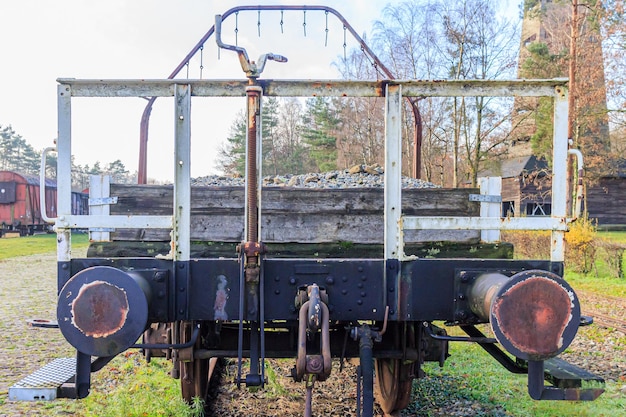This detailed image captures the rear view of a weathered, old-fashioned vehicle or piece of industrial equipment, prominently showcasing both metal and wood components. The bottom features heavy, train-like wheels, though it's not definitively on a track. The rear area includes a black bumper bar stretching horizontally, flanked by two metal cylinders and a hitch with a metal connection. A white metal guard rail rises up, and smaller chains or hooks dangle from a larger bar at the front. Steps protrude on either side for access. Rust patches hint at its age and the industrial setting. Surrounding the object is a farm landscape with green grass, brown soil, crops, trees, a distant barn, a silo, and a partly cloudy sky tinged with white and blue, contributing to the rustic atmosphere. The scene is devoid of people and text, emphasizing the focus on the object itself and its bucolic backdrop.